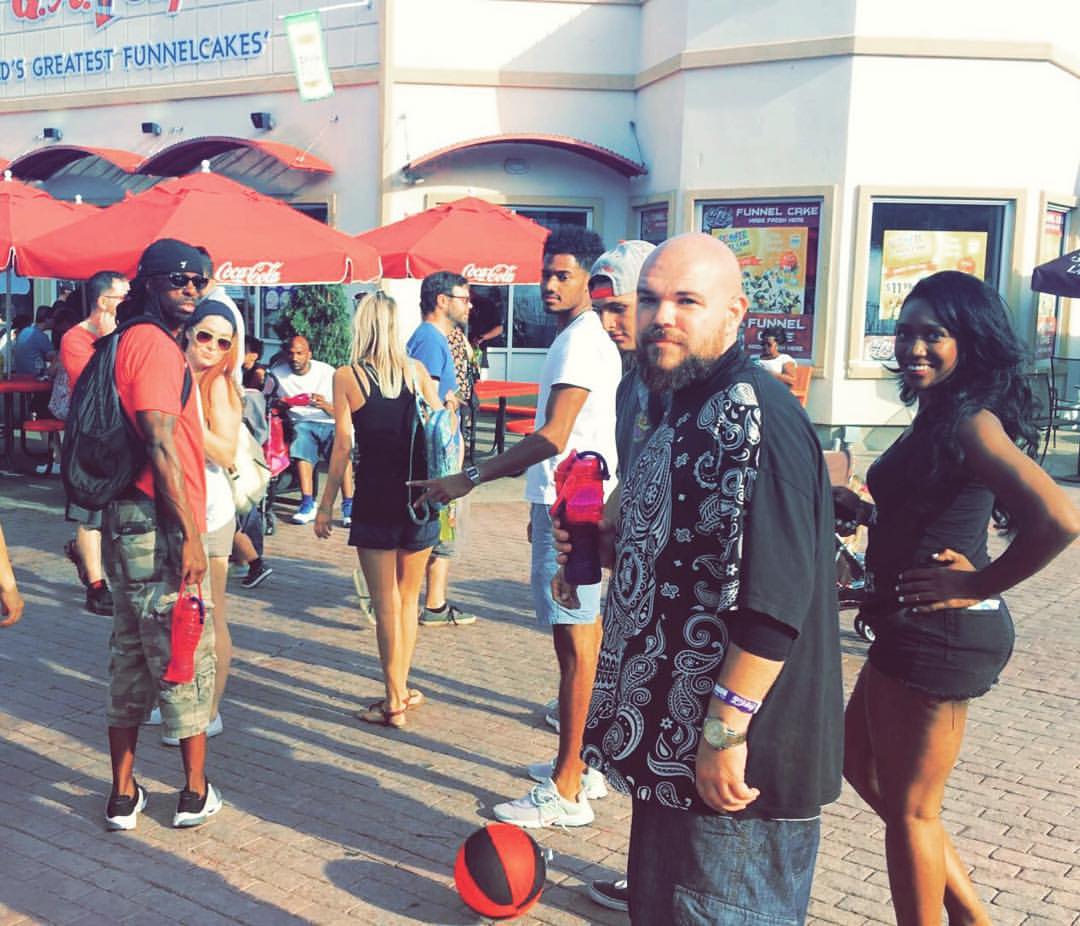A vibrant photograph captures a diverse group of people on a bustling sidewalk outside a stucco establishment famed for its funnel cakes. A large sign overhead reads "The World's Greatest Funnel Cakes" in blue lettering, with a prominent funnel cake poster below. The establishment’s name appears in red above the window adorned with white lettering advertising funnel cakes. The setting features several curved windowsills and three red Coca-Cola umbrellas shading red picnic tables, with a partially visible blue or black umbrella at the far right.

In the scene, an African-American man in a white shirt, jean shorts, and blue and white sneakers sits at a table, another man stands near him looking away, and another in a blue shirt and glasses walks by. A couple stands on the left; she, a white woman with red hair, a scarf, a blue bandana, sunglasses, and a hand resting on the chest of an African-American man in camo shorts, black do-rag, sunglasses, a red shirt, and holding a red water bottle.

A white woman with blonde hair and black tank top and shorts, stands next to another African-American man flashing a peace sign. Nearby, a person kicks a red and black soccer ball, wearing a backward baseball cap. Dominating the foreground, a bald, bearded man in a black shirt with paisley designs poses alongside various others, including an African-American woman in a black tank top and shorts, smiling with her hand on her hip. This lively gathering, characterized by its varied summer attire and communal atmosphere, encapsulates a joyous outdoor moment centered around a beloved local eatery.